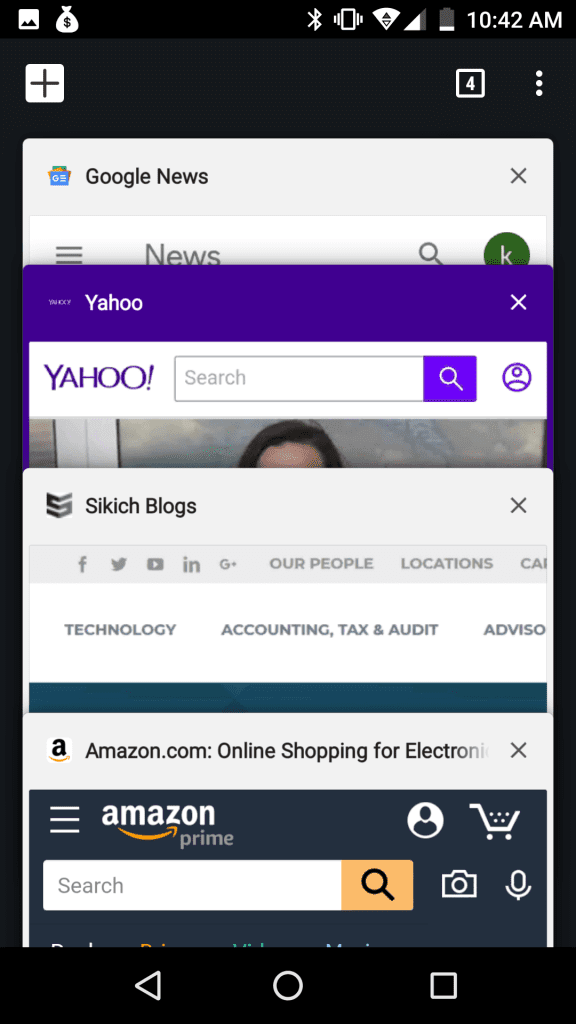The screenshot of the phone displays various elements in its user interface. In the top-left corner, there are two unfamiliar icons. On the upper right, common status icons are visible: Bluetooth, Wi-Fi with approximately 75% signal strength, and a battery icon showing less than 25% charge. The current time is 10:42 a.m. Below the status bar, a Google News app interface is partially visible. It features a magnifying glass icon for search and a green oval with a white letter 'K' inside. 

Underneath the Google News section, another window appears with a dark purple border at the top, labeled "Yahoo." It includes a search bar and a generic default profile picture. Beneath this, a light gray bar contains tabs labeled "Secrets," "Blogs," "Our People," "Location," "Technology," "Accounting," "Tax and Audit," and "Amazon.com Online Shopping for Electronics."